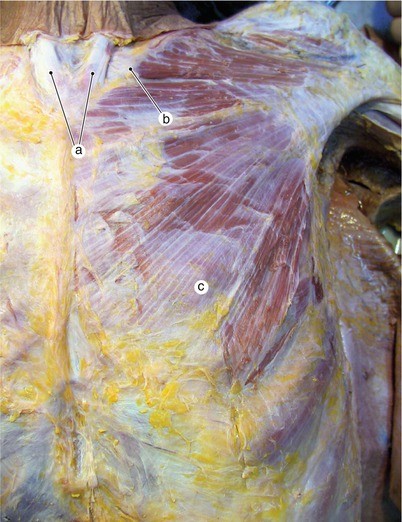This detailed photograph showcases the anatomical structure of the human chest with the skin meticulously removed to reveal the underlying muscles. The exposed muscles predominantly exhibit a reddish hue interspersed with intricate white lines, likely representing connective tissue or tendons. Central to the chest, and extending below it, are distinct yellowish sections, indicative of adipose tissue or fat deposits, accompanied by sporadic white areas that may denote additional connective or structural tissues. These color patterns are not confined to the chest alone but also extend to the shoulders.

The image focuses solely on the chest region, excluding any views of other body parts. Overlaying the photograph, precise annotations are visible, indicating edited lines and labels for educational or illustrative purposes. Near the neck, a black line extends upwards, culminating in a circled "A". Correspondingly, a similar black line on the right side ends with a circled "B", and another black line below the chest finishes with a circled "C". These labels, enclosed in small white circles, assist in identifying different segments within the chest anatomy, providing a clear and educational view of the musculature and associated tissues.